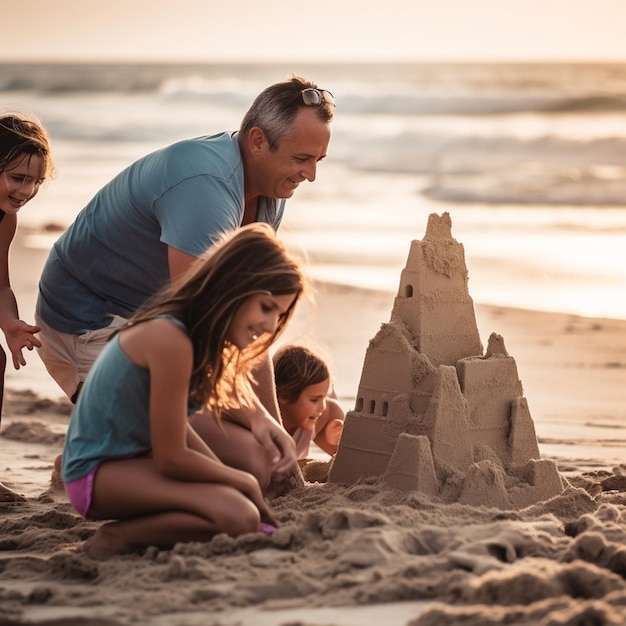In the bright, sunlit image, a joyful family is busy building an elaborate, multi-level sandcastle at the beach, near the water's edge with waves crashing in the background. The father, who has graying temples, glasses perched on his head, and is clad in a blue shirt and gray shorts, kneels beside the impressive triangular sandcastle adorned with little windows in its towers. Surrounding him are his three young daughters, all with long brunette hair, contributing smiles and laughter. One daughter, dressed in a blue shirt and pink shorts, is kneeling beside him, shoveling sand energetically. Another daughter’s head, with dark hair, is seen smiling just beside the sandcastle, while the youngest’s beaming face and tiny arm peek out from behind their father. The golden sand around them is dotted with holes and indents where the children have been digging eagerly under the brilliantly shining sun.